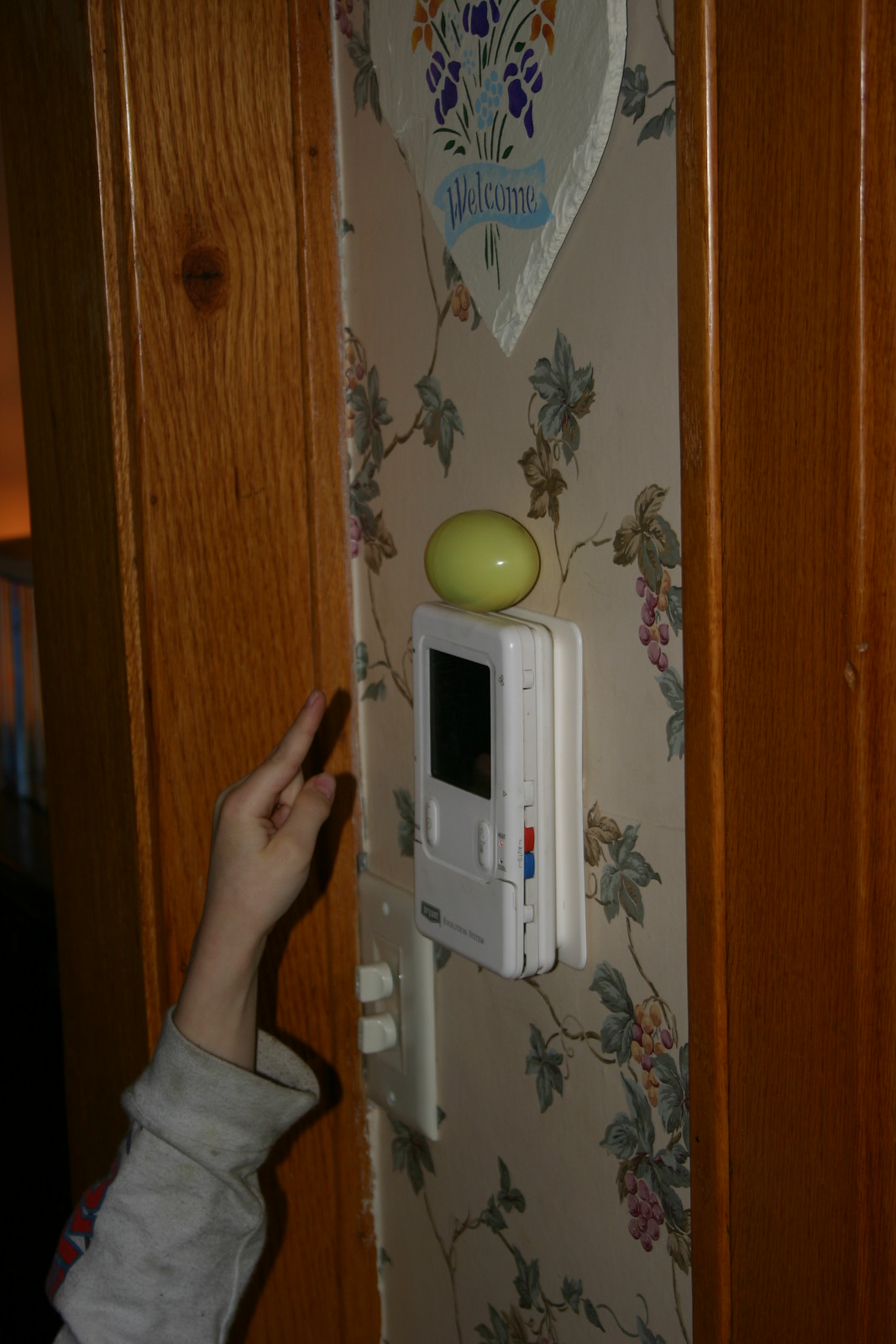In this photograph, a colorful Easter egg sits atop a Honeywell thermostat, which is mounted on a wallpapered wall adorned with a delicate vine pattern. To the bottom left of the thermostat, there is a light switch. A young person, dressed in a gray shirt, points at the yellow plastic egg, their finger close to the egg. Above the thermostat, a small, white heart decorated with flowers and a blue "Welcome" banner adds a charming touch. The thermostat itself is equipped with a red and blue switch on the right side. The wall is flanked by ornately crafted wooden moldings, likely made of maple-stained pine, framing the wallpapered section neatly. Small shrimp pieces are scattered incongruously, adding a quirky element to the scene.